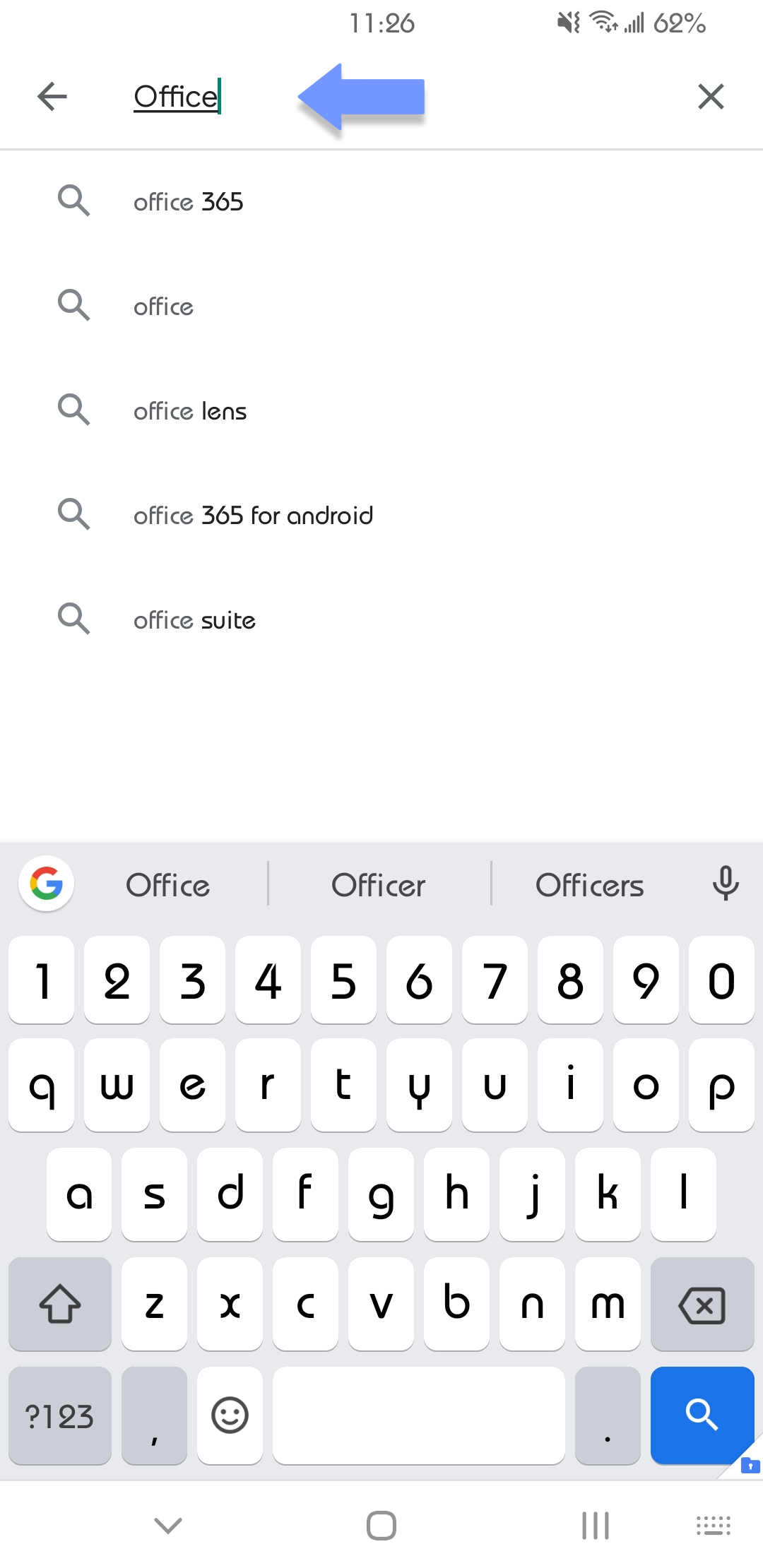This detailed screenshot showcases various elements of a smartphone interface, reflecting a search in progress. At the top, it indicates the time "11:26" alongside an icon suggesting the device is on silent mode, a Wi-Fi signal icon showing strong connectivity, and a battery level at 62%. The main background is white with gray text, featuring a heading labeled "office" accompanied by a blue arrow pointing to it. Below, a list of related search suggestions appears, each prefixed by a bright magnifying glass icon: "Office 365," "Office," "Office Lens," "Office 365 for Android," and "Office Suite." 

Further down, a gray keyboard is visible, showing a standard layout with off-white keys and black letters, numbers ranging from 1 to 0, and a gray microphone icon to the right. Above the keyboard, there's a white circle with the familiar red, gold, green, and blue Google logo, and search suggestions for "office," "officer," and "officers." At the very bottom lies a blue and white search icon. Additionally, an array of utility icons such as a down arrow, a square, lines, and a mini keyboard icon is aligned underneath the keyboard, enhancing the user's search spontaneity and functionality.